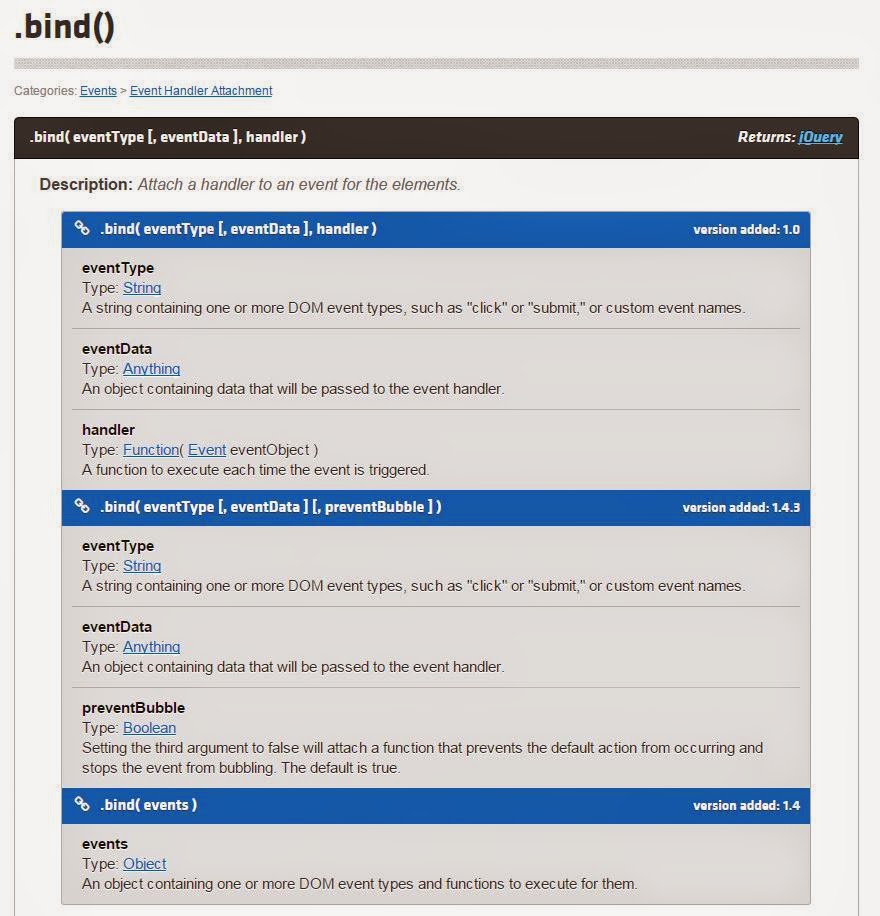The image features a detailed diagram set against a gray background, specifically focusing on the '.bind()' method in jQuery. Various elements of the diagram are highlighted in blue, adding visual distinction. The diagram is organized into categories and sections such as events and event handler attachment. 

A prominent black bar introduces the definition of '.bind()' with the syntax shown as: 

- `.bind( eventType, eventData, handler )`

This section explains that it returns a jQuery object and includes a brief description: "Attach a handler to an event for the elements".

Another section highlighted by a blue bar elaborates on the .bind() method, detailing its parameters:
- `.bind( eventType, [ eventData ], handler )`

Key terms like 'eventType', 'eventData', and 'handler' are highlighted in blue, indicating their significance. Additional information provided includes:
- Version added: 1.0
- Event type: Type specified as either 'string' or 'setting' in blue
- Event data: Type specified as 'anything' in blue
- Handler type: Function (highlighted in blue), with 'event' and 'event object' also denoted in blue.

Furthermore, another blue-highlighted section specifies:
- `.bind( eventType, [ eventData, preventBubble ] )`

Here, it is noted that this form of the method was added in version 1.4.3.

Overall, the image serves as a comprehensive guide on the syntax, parameters, and use cases of the '.bind()' method in jQuery.